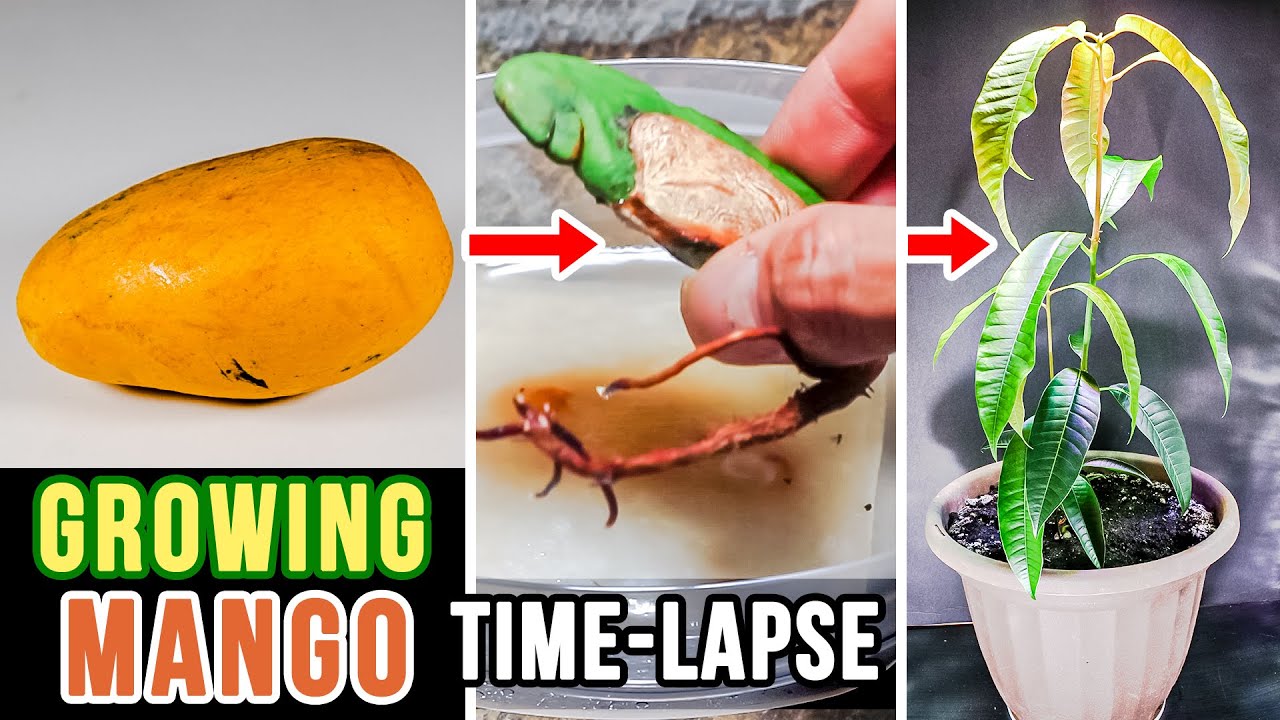A horizontally oriented image features three realistic photographs set side-by-side in distinct sections. The left section showcases a yellow-orange mango with a text box at the bottom that reads "Growing Mango," using yellow and green font for "Growing" and orange font with a white border for "Mango," all on a black background. A red arrow points from this section to the middle one, which displays someone holding a partially green mango seed with emerging roots. This middle section also has a text box at the bottom that says "Time-Lapse" in bold white font on a black background. Another red arrow directs from the middle to the rightmost section, which depicts a white flower pot filled with dirt from which a green mango plant is sprouting. The entire image is set against a gray background.